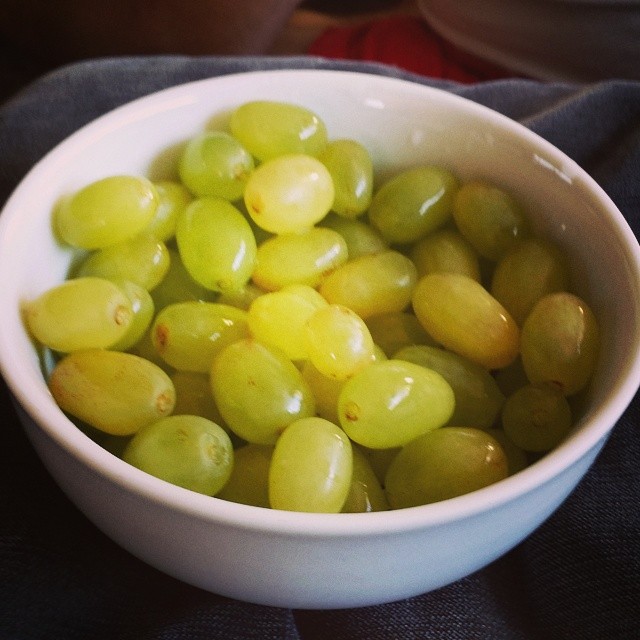A slightly blurry photograph captures a white, shiny ceramic bowl filled with freshly washed green grapes on a textured, grayish fabric. Most grapes are a typical oval shape, displaying a mix of green shades, with some exhibiting a yellowish tint or a subtle purplish hue. Brown specks mark where the grapes were attached to the vine. Water droplets glisten on both the grapes and the bowl, reflecting light from the upper right. The bowl seems nestled in the fabric possibly on a wooden surface. A hint of red and a wooden plate are visible in the top corner, though the background details are fuzzy and indistinct.